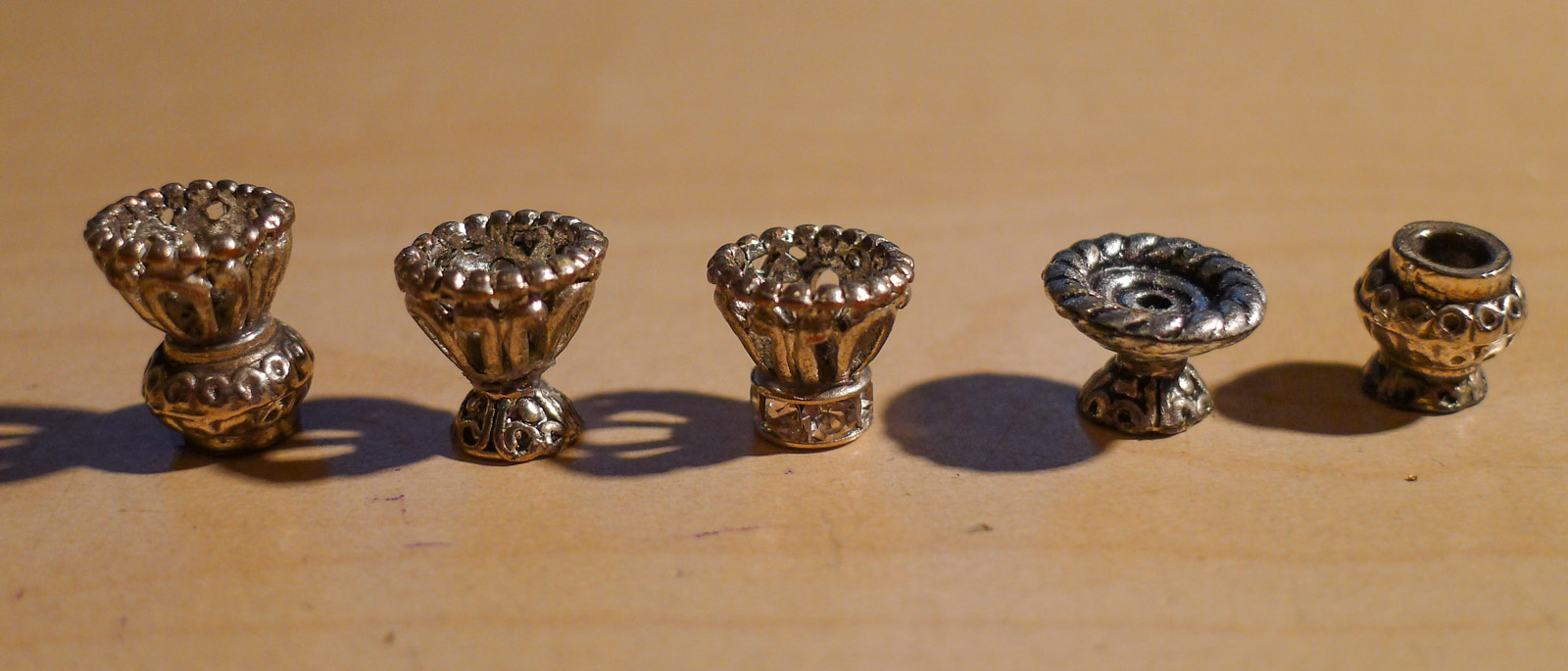This photograph captures a striking assortment of five antique doorknobs or ornamental knobs, meticulously arranged on a light honey-toned wooden surface, accentuated by darker streaks. The knobs vary in design, size, and color, with four showcasing a rich, brownish-copper hue, while the fifth stands out in an elegant silver. Each knob features intricate swirly or circular patterns, highlighting their handmade craftsmanship. The first knob resembles a pineapple and is golden. The second transitions from a round top to a triangular base, also in gold. The third knob has a round top that tapers inward before expanding into a ringed base, and is golden as well. The standout silver knob has a round top, narrows to a slim middle, then broadens again at the bottom. The final gold knob appears to be upside down, revealing the screw ring. All the knobs cast subtle shadows to their left, adding depth to the scene. The variations in design and color suggest a collection of unique, antique drawer knobs, each telling its own story.